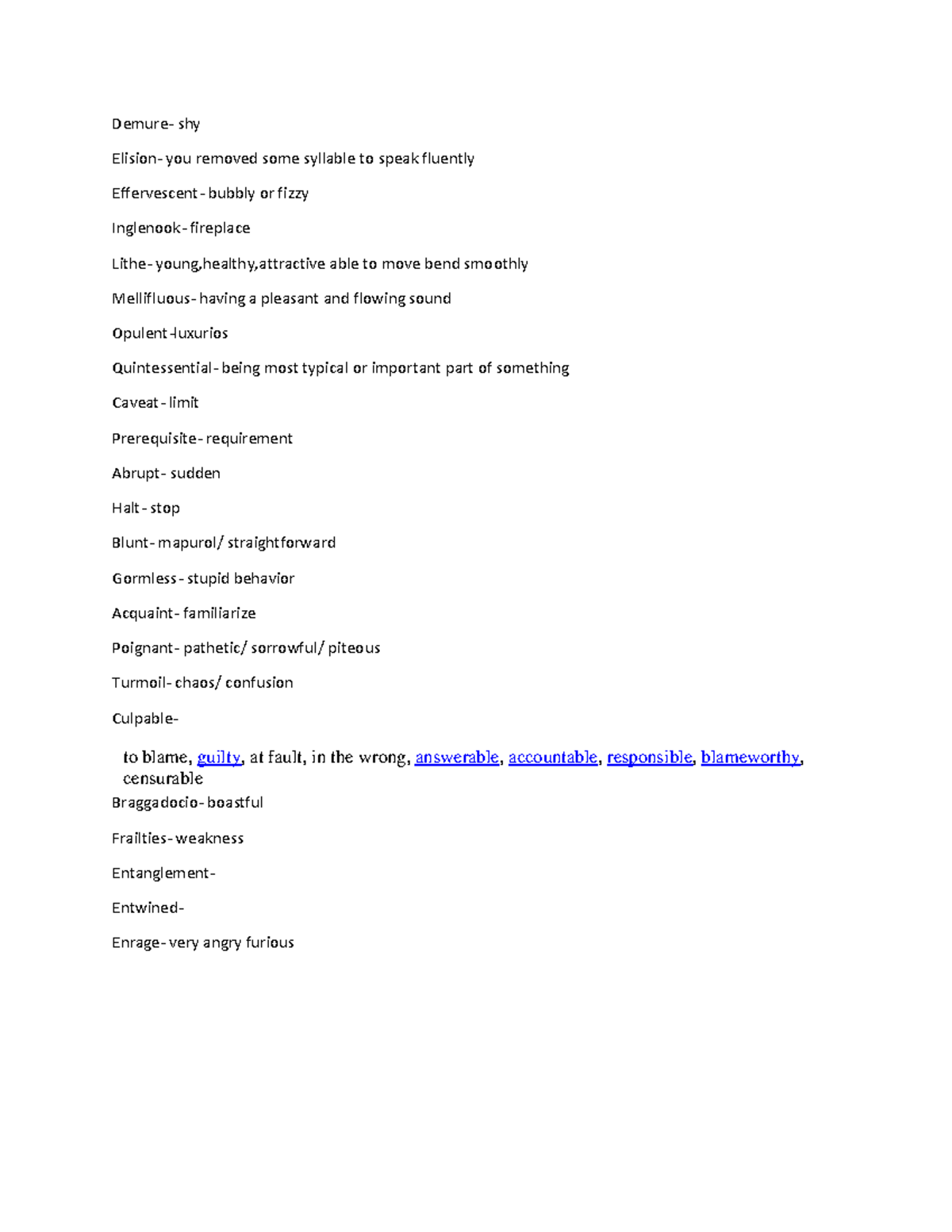The image displays a white background adorned with a collection of words in blue, each accompanied by a brief definition. However, certain words and phrases stand out in red or are underlined for emphasis. The words are as follows:

1. **Demure**: Shy.
2. **Elision**: The act of removing some syllables to ensure fluent speech.
3. **Effervescent**: Bubbly or fizzy.
4. **Ingle nook**: Fireplace.
5. **Lithe**: Young, healthy, attractive, able to move or bend smoothly.
6. **Melliferous**: Producing or full of honey; pleasantly flowing.
7. **Opulent**: Luxurious.
8. **Quintessential**: Representing the most typical and important example of something.
9. **Caveat**: A warning or condition.
10. **Prerequisite**: A required condition; something that must be fulfilled beforehand.
11. **Abrupt**: Sudden.
12. **Halt**: Stop.
13. **Blunt**: Straightforward, often to the point of being impolite.
14. **Bluntness**: The quality of being straightforward, sometimes perceived as stupid behavior.
15. **Acquaint**: To familiarize.
16. **Poignant**: Evoking a sense of sadness or regret; sorrowful, piteous.
17. **Turmoil**: A state of chaos and confusion.
18. **Culpable**: To blame, guilty, at fault, in the wrong (this is underlined in blue).
19. **Answerable**, **Accountable**, **Responsible**, **Blameworthy**: These four words are underlined in blue indicating the emphasis on their meaning as synonyms of culpable.
20. **Censorable**: Deserving of censure or criticism.
21. **Braggadocio**: Boastful or arrogant behavior.
22. **Fertility**: Initially misunderstood, it indicates the capacity for reproduction, but here it is dubbed as **weakness**.
23. **Entanglement** and **Entwined**: Presented without definitions but likely suggesting being involved in complications or intricate involvement.
24. **Enraged**: Very angry, furious.

Each term is distinctly separated, with underlined words and color differences accentuating the importance of particular words. The precise and thorough definitions provided aid in understanding each term in depth.